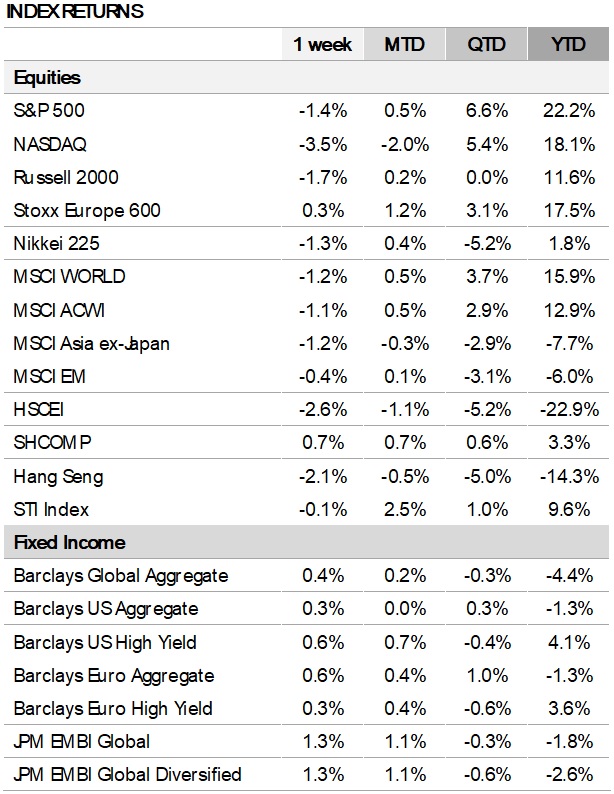The image features a detailed financial chart with a clean, white background. At the top left corner, the title "INDEXED RETURNS" is prominently displayed in bold, dark black uppercase letters. Below the title, there is a timeline represented by a horizontal progression of color-changing segments. The timeline transitions from white at the start, through light gray in the middle, to darker shades of gray towards the right. Each segment is labeled in black capital text: "ONE WEEK" (with the numeral '1' and the word 'WEEK'), "MTD" (Month-To-Date), "QTD" (Quarter-To-Date), and "YTD" (Year-To-Date).

On the left side of the chart, there are two main categories: “EQUITIES” and “FIXED INCOME.” Under the “EQUITIES” section, a list of various stock indices is presented, each in a separate row. These are:

- S&P 500
- NASDAQ
- Russell 2000
- Stoxx Europe 600
- Nikkei 225
- MSCI World
- MSCI ACWI
- MSCI Asia ex-Japan
- MSCI EM
- HSCEI
- SHCOMP
- Hang Seng
- STI Index

Below the “EQUITIES” section, the “FIXED INCOME” category is marked by a gray banner with its title in bold, capitalized letters. Under this category, the list includes different Barclays and JPM fixed income indices:

- Barclays Global Aggregate
- Barclays US Aggregate
- Barclays US High Yield
- Barclays Euro Aggregate
- Barclays Euro High Yield
- JPM EMBI Global
- JPM EMBI Global Diversified